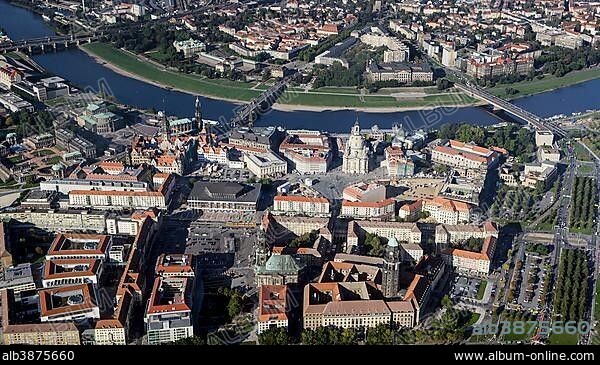This is a high-resolution, color aerial photograph of an unidentified city featuring a densely built urban landscape with numerous closely-packed buildings predominantly adorned with red roofs. The cityscape, captured from an aircraft or drone, includes a prominent waterway, likely a river or a lake, that divides the settlement into two distinct sections. The waterway is connected by three visible bridges, linking the main urban area in the foreground with a smaller, somewhat circular landmass in the background. This back section appears greener with patches of trees and grassy areas along the riverbank. Prominent features in the photograph include a church tower and clusters of white buildings, likely constructed from a distinctive type of stone. The photograph, edged in black at the bottom, bears the watermark 'Album' and the URL 'www.album-online.com' alongside the identification number 'ALB3875660'.